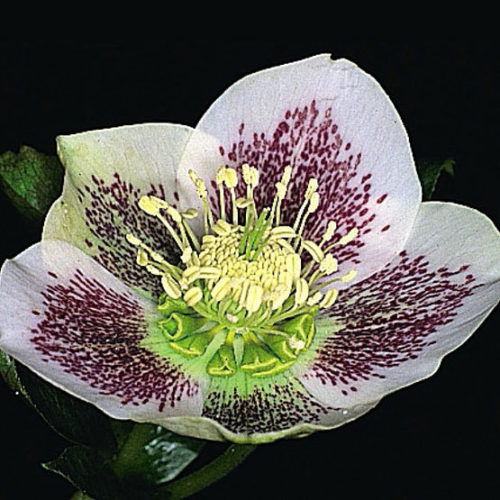This image features a close-up of a hellebore flower, otherwise known as a lenten rose, captured in a square, approximately four-by-four-inch photograph. The flower is centrally positioned, with its large petals extending outward, some slightly bowled at the edges. The petals are predominantly white, with a maroonish-red speckling concentrated towards the center, creating a visually striking contrast. One petal on the upper left has a noticeable green tinge. The photograph’s background is pitch black, likely achieved using a flash, rendering it impossible to determine whether the setting is indoors or outdoors.

The focus of the image is the intricate details of the flower's center. At the base of the flower's core is a green area, from which slender tubes, green with vibrant yellow tips, emerge. Encircling these are the stamens—rounded bunches with light yellowish cream elongated ends. The vibrant yellow of these stamens adds to the flower's allure. Beneath the flower, a dark stem with equally dark, waxy leaves extends from the lower left, adding depth to the composition. The photo appears somewhat noisy and pixelated, suggesting it might be a low-resolution image that's been digitally enhanced.